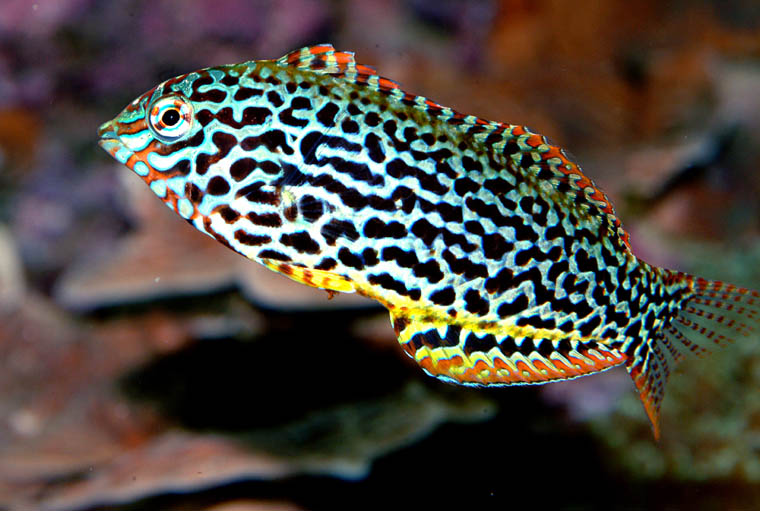The image depicts a striking close-up of a small, tropical fish swimming slightly upright to the left in an aquatic environment. The fish, positioned centrally against a subtly hued backdrop featuring shades of pink and orange, likely suggests the presence of coral, indicating a saltwater habitat. The fish's elongated, torpedo-shaped body flaunts a captivating marbled pattern with a predominantly black and blue body interspersed with silver and white. Distinctively, the fish's left side is visible, showcasing vibrant orange and yellow accents. 

Its body is predominantly black with intricate blue and silver zebra-like patterns. The top of the fish features a bright orange outline with hints of silver, while the dorsal fin extends from the tip of its neck to the tail, adorned with orange marbling. The pectoral fin is small, whereas the abdominal fin near the tail is larger and highlighted with yellow and orange pigments. The fish’s translucent tail fin, also tinged with blue and orange, adds to its finesse.

Notably, the fish's face is a mosaic of orange, silver, and black, with a striking eye that is blue at its center encircled by white and orange. The detailing around the eye speaks to the intricate beauty of the fish, affirming its possible species as a distinctive and vibrant tropical variety.